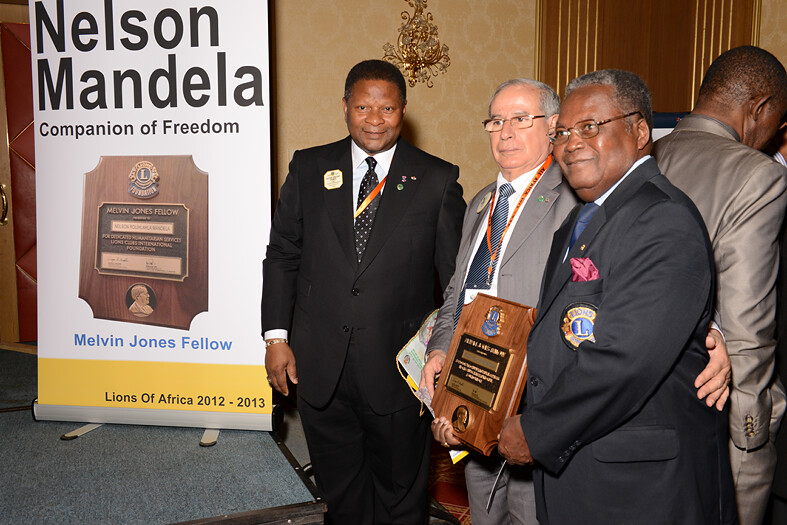In an elegant room adorned with brown wood panels and gold embellishments, a group of men stands next to a stage, engaging in a significant moment of recognition. The central figure, a black man in a sophisticated black suit, holds a plaque, joined by another black man in a dark suit to his right and a white man in a light gray suit with a blue tie to his left. Behind them, another black man in a light gray suit stands with his back to the camera, partially turned towards the group.

The stage itself features a prominent poster with the heading "Nelson Mandela, Companion of Freedom." Beneath this title, the same plaque now held by the central figure is displayed, which reads "Melvin Jones Fellow." At the bottom of the poster, a yellow rectangle marks the honored timeframe, stating, "Lions of Africa 2012-2013."

This photo captures an awarding ceremony moment where the prestigious Melvin Jones Fellow plaque is being presented as part of a tribute to Nelson Mandela's legacy. The attendees, all wearing name-tag lanyards, add to the ceremonial atmosphere as they pose for what appears to be a photo opportunity, highlighting an event steeped in recognition and respect.